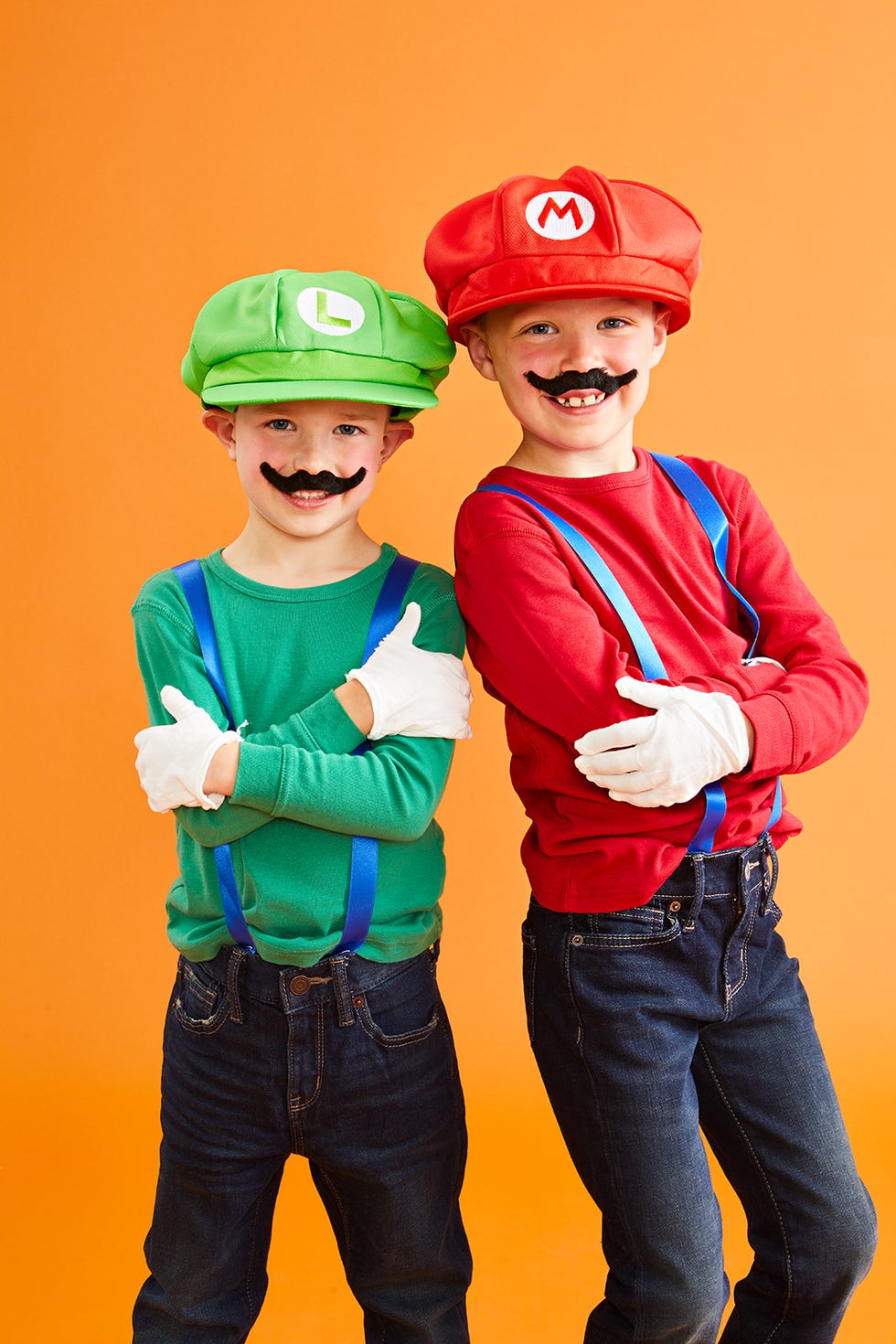In the image, set against a gradient orange wall that shifts from darker orange in the top left to lighter orange in the bottom right, stand two boys dressed in detailed Super Mario Brothers costumes. The taller boy on the right is dressed as Mario, donning a red hat emblazoned with a white circle and red "M", a red long-sleeved shirt, white gloves, blue suspenders, and dark blue jeans. His outfit is completed with a fake black mustache placed above his lip. Next to him, the shorter boy portrays Luigi, wearing a green hat with a white circle featuring a green "L", a green long-sleeved shirt, white gloves, blue suspenders, and dark blue jeans. He, too, sports a similar mustache. Both boys strike a pose with arms crossed—Mario leaning slightly on Luigi, capturing a moment of playful camaraderie against the vivid backdrop.